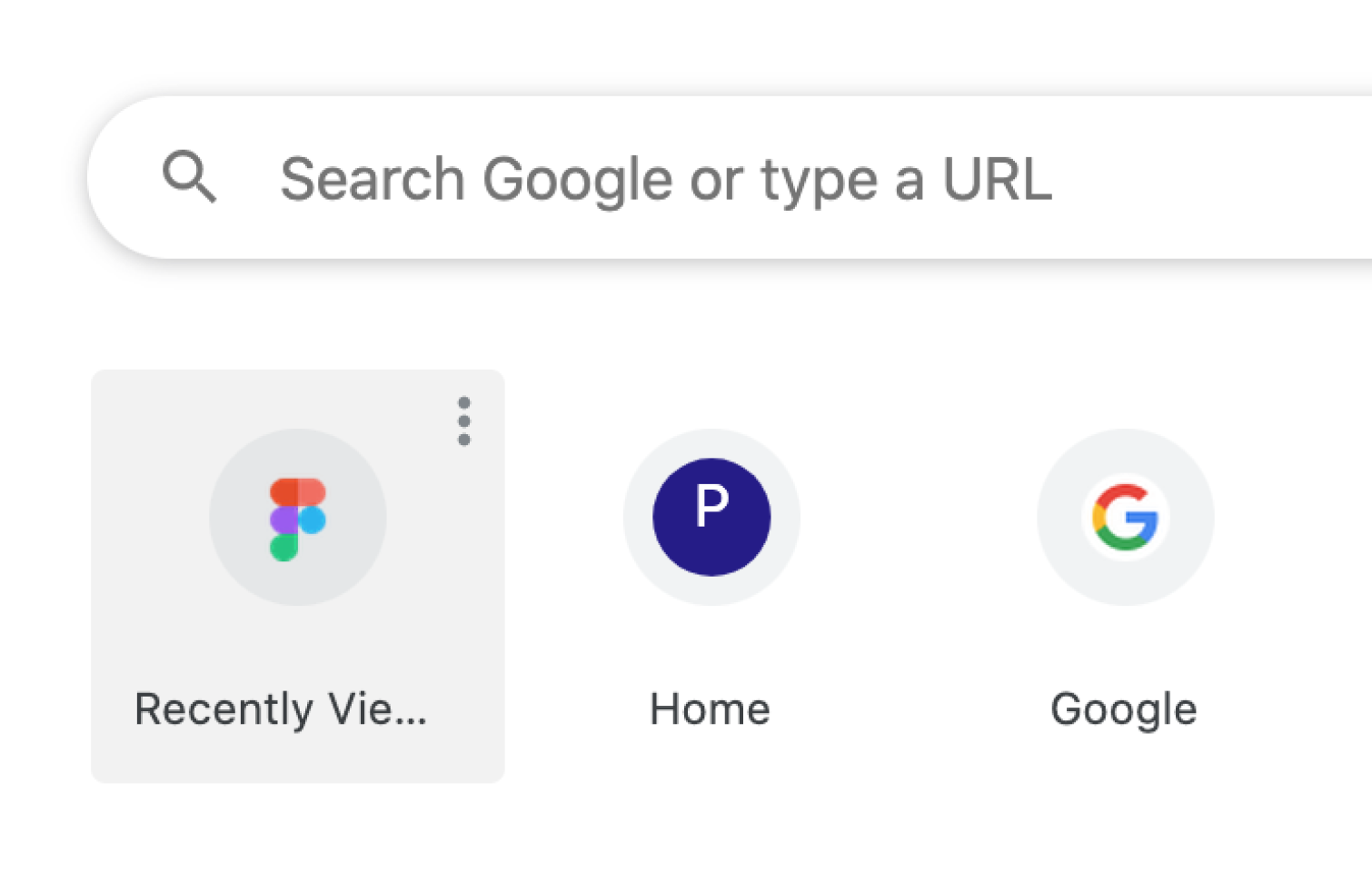In this image, the background is white, with the primary focus being on a visually structured interface. At the top, there is an elongated oval outlined in grey, housing a grey magnifying glass icon on the left side. Beside the icon, the text "Search Google or type a URL" is displayed in grey font.

Below this oval section, there is a light grey box containing a vertical alignment of circles. The first row has a grey circle with three vertical dots inside, adjacent to a red circle and an orange circle. Directly below this row is a purple circle and a blue circle. Following that, towards the bottom of this section, there is a green circle on the left side. Below these circles, in black font, the text "Recently viewed" is displayed with three horizontal dots following it.

In the next section, the background remains white. Here, there is a grey circle and a blue circle containing a white letter "P." Underneath, the word "Home" is written in black font.

The final section features another grey circle with the Google logo, characterized by colors red, orange, green, and blue forming the letter "G." Beneath this logo, the word "Google" is printed in black font.